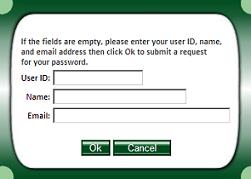This image is a screenshot of a login page with a modern and clean design. The background is a solid green color, providing a fresh and calming aesthetic. Centrally positioned on the page is a rounded white rectangle containing form elements and instructional text.

At the top of this white area, a clear instruction reads: "If the fields are empty, please enter your User ID, name, and email address, then click OK to submit a request for your password." 

Directly below this text, there are three individual input fields aligned vertically, each designated for entering the User ID, name, and email address, respectively. Each field is outlined in a thin border for better visibility.

Below these input fields, there are two green buttons, centered within the white rectangle. The left button is labeled "OK," and the right button is labeled "Cancel," both in clean white text. The buttons stand out against the white background, inviting user interaction.

Encapsulating the white rectangle is a thin black outline, which further distinguishes it from the green background, adding to the overall clarity and organization of the page's layout.